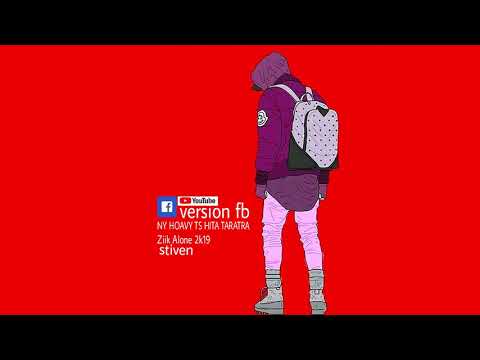In this vibrant red background, a young girl stands with her back turned slightly to the right, attired in a purple jacket with the hood up, revealing a matching purple shirt that drapes below her hips. She wears light pink pants and gray ankle-high boots. A black and white badge is visible on her left upper arm of the jacket. Her gray and black backpack is slung over her shoulders, and she tops off her outfit with a purple hat. She gazes downward at a banner in front of her that prominently features a YouTube logo, a Facebook symbol to the left, and white text reading "Version FB." Below this are the letters "N-Y-H-O-A-V-Y-T-S-H-I-T-A-T-A-R-A-T-R-A," followed by "Z-U-K ALONE 2K19" and "S-T-I-V-E-N." The image is framed by black rectangular strips at the top and bottom, adding a border to this digitally created or painted scene.